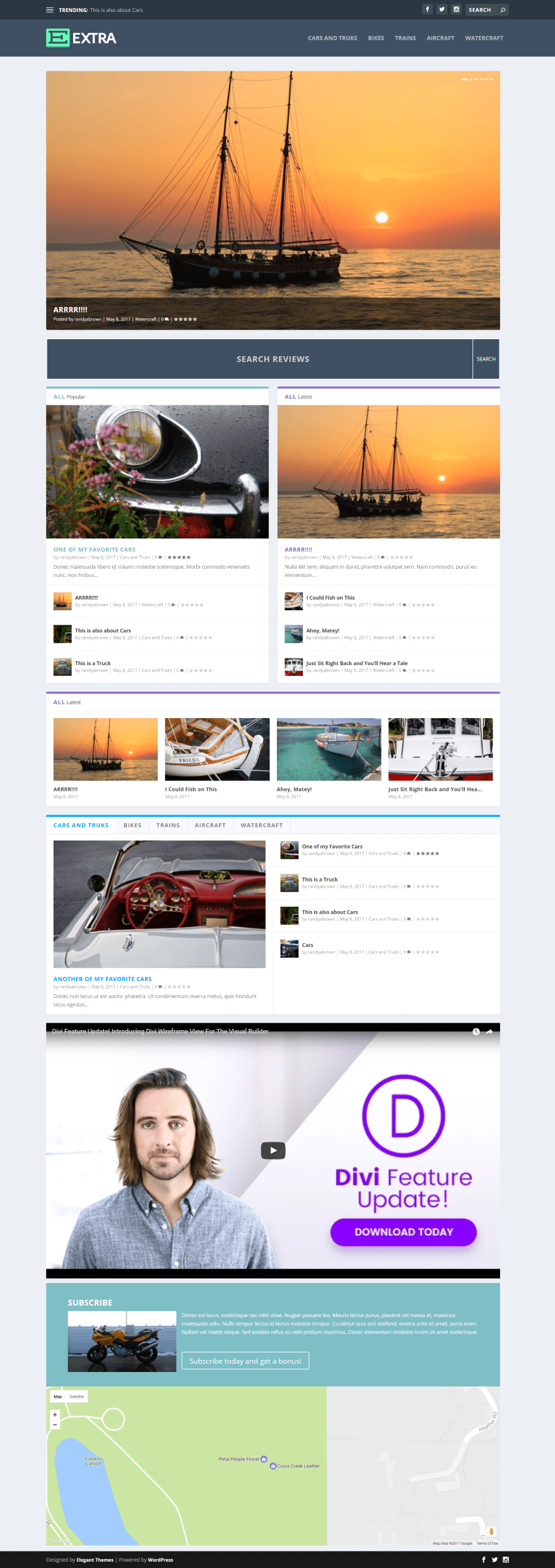In the image, we can see a screenshot of a website's homepage. At the top left corner, the website name "Extra" is prominently displayed in white text next to a green square logo featuring a large white "E." On the top right, three social media icons are visible: Twitter, Facebook, and LinkedIn.

Further down, a large squared image depicts a ship sailing on the sea with an orange-tinted sky in the background, giving the scene a dramatic and warm ambiance. Below this main image, there are two smaller boxed images: one on the left displays a vibrant flower, while the one on the right mirrors the earlier image of the ship.

In the bottom half of the image, a paused video screen shows a man with a fair complexion and dark brown hair. To the right of the video, the words "Divi Feature Update" are displayed, accompanied by a circular logo with a purple "D" inside it. Below this, a purple bubble with white text reads "Download Today," indicating a call to action.